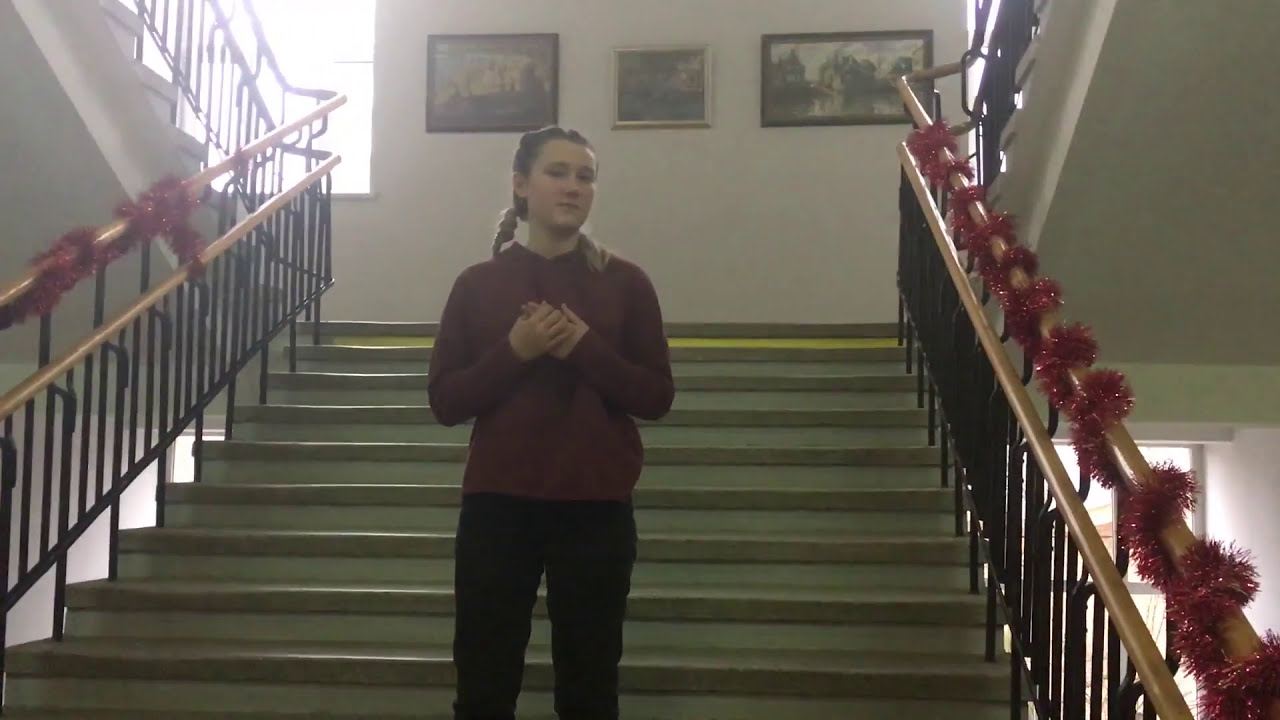In this dimly lit indoor photograph, a young brunette woman, likely in college, stands on a staircase with her hands clasped to her chest. She wears a long-sleeve maroon shirt and black pants, with her hair styled in French braids. Her cautious expression is subtly directed towards the camera, though slightly off to the side. The staircase features handrails wrapped in red holiday-style wreaths, suggesting a festive atmosphere. Behind her, a white wall displays three paintings: the left and right framed in black, and the center in gold. The setting's detailed colors include gray, yellow, red, black, white, tan, light brown, dark brown, and gold, creating a warm yet cautious ambiance.